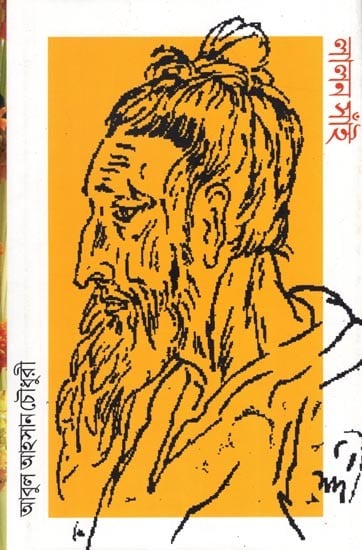This image appears to be the cover of a book and features a detailed, hand-drawn sketch of a man rendered in black lines. The man, who may be of Asian descent, is shown in profile, facing the left side of the image. He has a long, pointed nose angled downward, a pronounced beard, and a mustache extending from his short hair, which is tied up in a bun resembling a top knot. His expression is sad, with downcast eyes and a furrowed forehead, giving him a tired and weathered appearance. He is dressed in a garment with a V-neck collar, though the drawing only extends to about chest level. The background of the image is primarily orange, with some white areas. Foreign language text can be seen in red in the top right corner and in black in the bottom left corner. The image also includes an illegible signature in the bottom right corner.